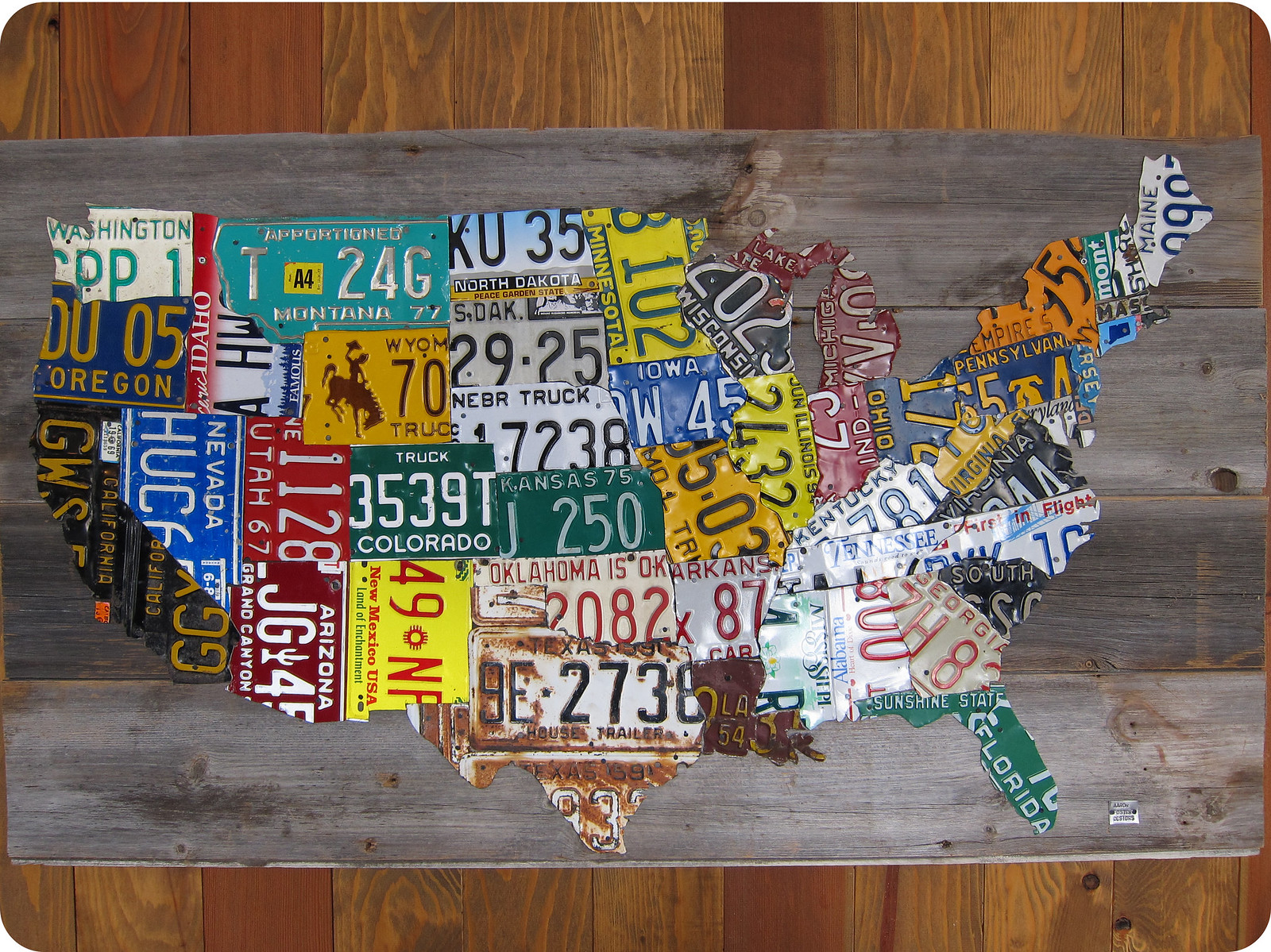The image depicts a highly detailed and creative piece of folk art resembling a map of the United States, meticulously crafted from license plates specific to each state. Each state is represented by a section of a real license plate cut precisely to match the state's shape. For instance, Maine's plate, with barely visible numbers, fits perfectly into the outline of Maine, while New York's plate displays part of the word "Empire," and the distinctive shape of Texas is recreated using two plates. Pennsylvania, New Jersey, California, Oklahoma, and Georgia are similarly represented, with Oklahoma's plate even reading "OK." The entire U.S. map, from Washington State in the northwest to Florida in the southeast, is set against a rustic backdrop of barn wood for a cohesive and artistic presentation. This detailed and impressive montage uses the authentic license plates from each state, enhancing its visual appeal and craftsmanship.